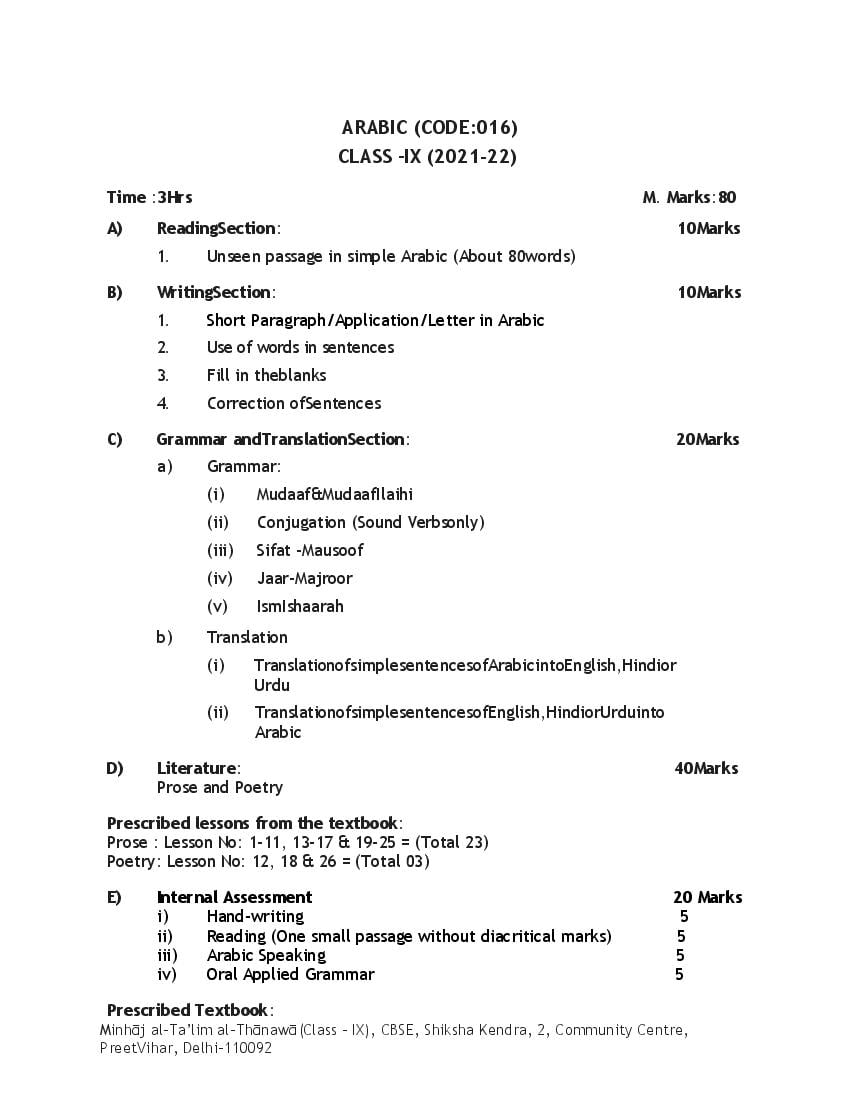This image is a detailed photocopy or printout of an educational syllabus, appearing as a high-quality, well-centered, and neatly spaced text document in black and white. At the top, in bold letters, it reads "ARABIC (CODE: 016) CLASS-IX (2021-22)," indicating it's for a Class IX Arabic course. The exam duration is specified as "Time: 3 hours," and "Marks: 80" is written to the right.

The syllabus is structured into distinct sections:

1. **Reading Section (10 Marks):**
   - It involves one unseen passage of about 80 words in simple Arabic.

2. **Writing Section (10 Marks):**
   - Tasks include writing a short paragraph/application letter in Arabic, using words and sentences, filling in the blanks, and correcting sentences.

3. **Grammar and Translation Section (20 Marks):**
   - This section comprises various subtopics like grammar (including Mudaf and Mudaf Ilayh, conjugation of sound verbs), Sifat-Mausoof, Jarr-Majroor, and Ism-Ishara. Translation tasks involve converting simple sentences between Arabic and English, Hindi, or Urdu.

4. **Literature Section (40 Marks):**
   - It covers prose and poetry lessons from the prescribed textbook "Minhoj al-Talim altonawa," including prose lessons 1 to 11, 13 to 17, and 19 to 25, totaling 23 lessons, and poetry lessons 12, 18, and 26, totaling 3 lessons.

5. **Internal Assessment (20 Marks):**
   - This includes handwriting (5 marks), reading a small passage without diacritical marks (5 marks), Arabic speaking (5 marks), and oral applied grammar (5 marks).

The prescribed textbook is from CBSE Shiksha Kendra, located at Community Center, Preet Vihar, Delhi-110092. The entire document exudes formality and is clearly intended for academic use, serving as a comprehensive guideline for the course's performance evaluation.